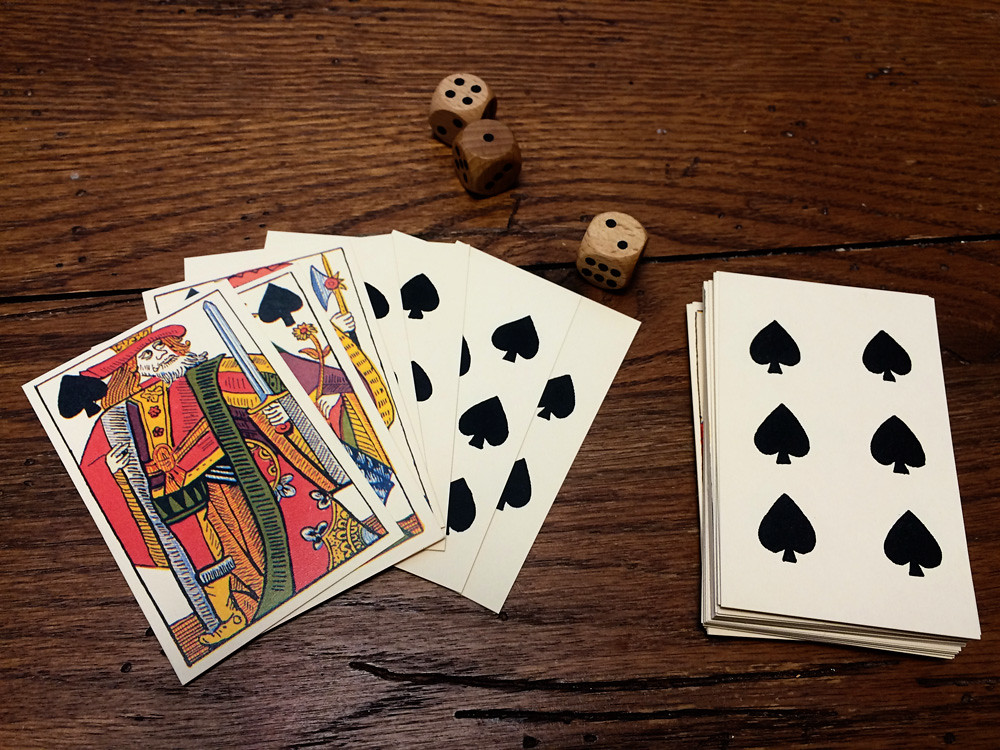The image features a slightly wider-than-tall layout, approximately 20% wider, displayed against a dark wood surface. The wooden background shows a distinctive division between two of the boards at around 60% up on the left side, aligned horizontally with the wood grain.

Prominently in the foreground are three dice positioned at the center top. They display the numbers four, one, and two respectively. Notably, the die showing one is quite dirty, with a grayish hue, while the other dice have mild dirtiness.

On the left-hand side, there is a collection of playing cards. The cards do not bear numbers, implying they are standard playing cards with only pictures and shapes. The foremost card is the Jack of Spades, depicted holding a sword, dressed in a long robe, and without a crown. The upper left corner features the spade symbol. The second card is partially visible, showing a figure associated with spades, distinguished by a spade symbol in the upper right corner. The third card shows a figure holding an axe, though the suit symbol is obscured.

Further to the right, there is a sequence of spade cards numbered one, two, three, and four. Adjacent to these is a separate stack topped by a six of spades card.